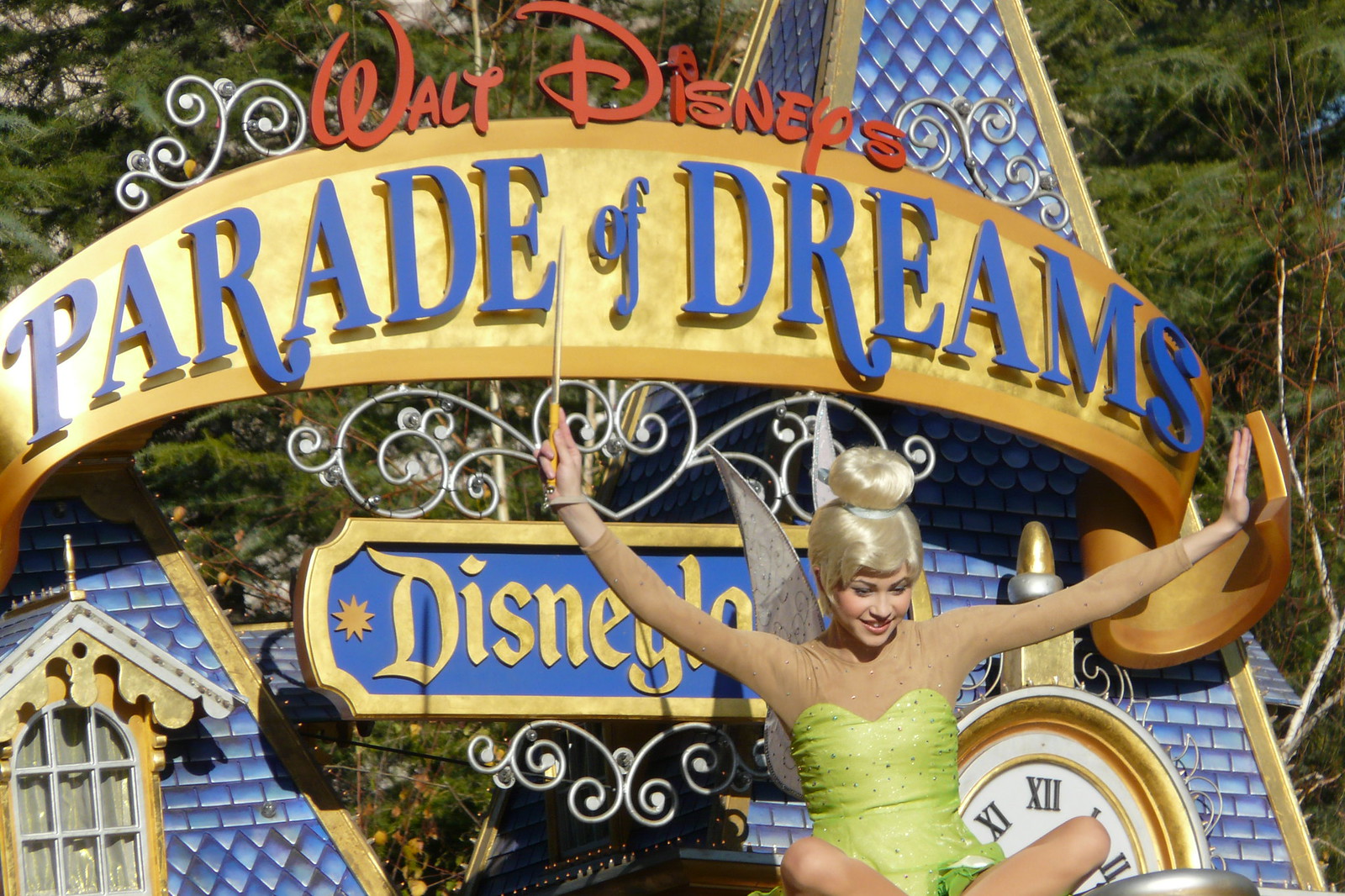This photograph captures a vibrant scene from the Disneyland Parade of Dreams, featuring a performer dressed as Tinkerbell. She sits cross-legged atop a parade float, dazzling in a green dress with a sweetheart neckline and fairy wings adorning her back. Her blonde wig is styled into a bun, and she has a radiant smile with her arms raised joyfully. The float is positioned in front of the iconic Disneyland castle, which prominently displays the signage, "Walt Disney" above "Parade of Dreams" and "Disneyland." The backdrop includes lush trees, enhancing the fairy-tale ambiance. Noteworthy details include the actress’s pantyhose-like arm coverings, her makeup, and a wand held in her right hand, which is on the left side of the picture. The photograph, taken during the day, beautifully captures the magic and grandeur of this Disneyland spectacle.